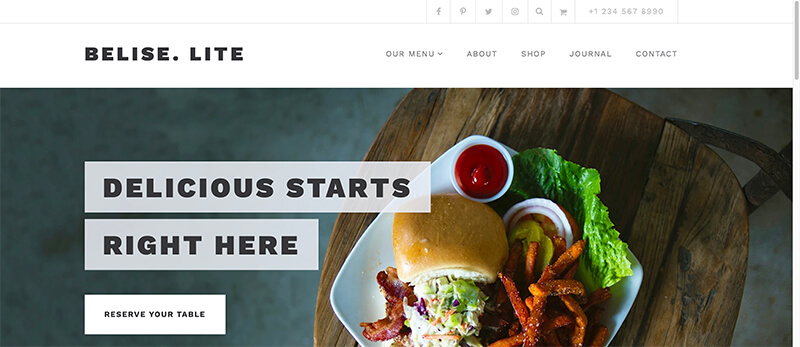The image captures a detailed view of a webpage for BELISE LITE, with "BELISE" spelled "B-E-L-I-S-E" followed by a period, and "LITE" spelled "L-I-T-E," both in bold, black, all-capital letters positioned at the top of the page. To the right of the webpage's header, there's a drop-down menu offering navigation options labeled as "About," "Shop," "Journal," and "Contact." Above the navigation, social media icons are displayed, and the company's phone number is also visible.

In the central portion of the webpage, there's an appetizing image of a meal served on a plate. The meal appears to include a green lettuce leaf, a cup of ketchup, coleslaw, and a buttered biscuit. The main dish appears to be either lobster or french fries, possibly sweet potato fries given their orange hue. There also seems to be strips of bacon enhancing the meal's visual appeal. Over the image, in white boxes with black text, the tagline "Delicious starts right here" is prominently displayed, accompanied by a clickable button labeled "Reserve Your Table."